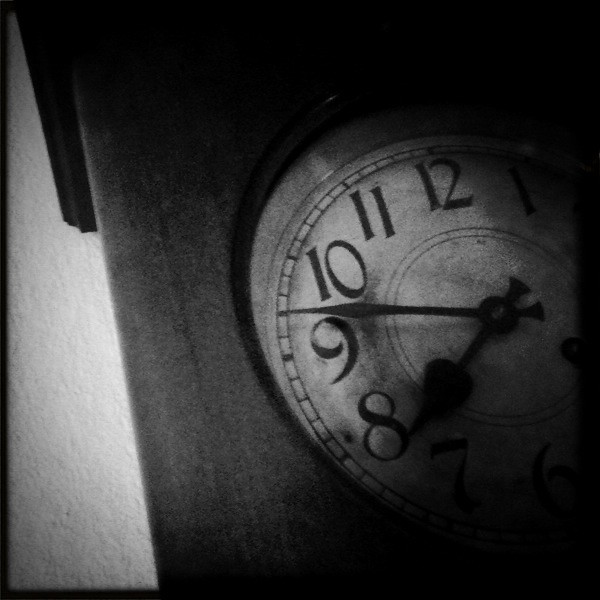A monochromatic black-and-white photograph captures the elegant charm of a vintage grandfather clock. The image focuses on the front half, particularly highlighting the clock face. The small hour hand, with its thicker, distinctive black arm, points towards the number 8, while the slender minute hand, tapering into a sharp point, is positioned between the 9 and 10. The clock itself is crafted from dark wood, exuding a timeless sophistication. Behind the clock, a light-colored wall with a drywall texture provides a subtle, contrasting backdrop that enhances the clock's prominence in the frame.